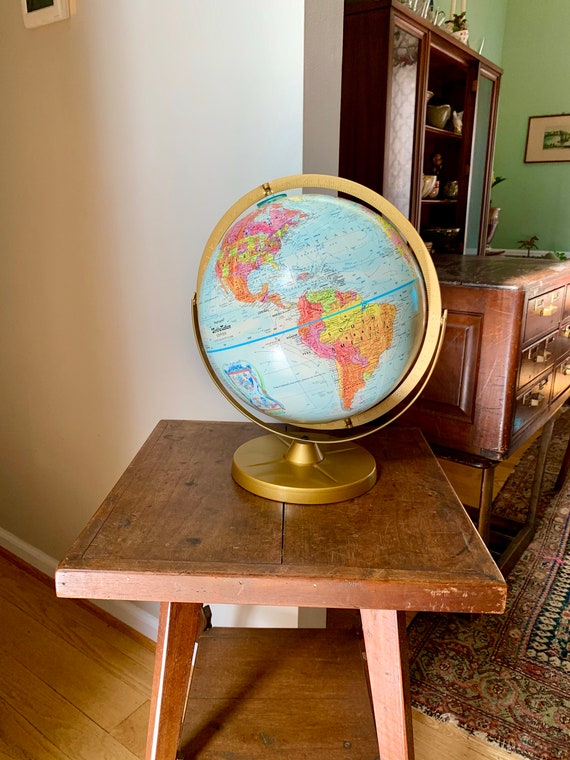In this detailed photograph of an interior space, we observe the meeting point between two distinct rooms. To the left, there is a hallway defined by a clean white wall, while to the right, a room with light green walls can be discerned, showcasing a large wooden hutch with multiple drawers and glass-fronted upper shelves. Central to the composition is a vintage wooden table characterized by its tapered legs and a two-board top with wood trim. This table, placed vertically, holds an intricately designed globe. The globe features a gold circular base and a gold meridian ring. Its surface prominently displays the blue of the oceans, along with the intricately colored continents of North America, Central America, and South America. The flooring beneath the table is wooden, complemented by a faded Persian-style rug located in the bottom right corner. The image offers a glimpse into a cozy, well-decorated home interior, merging classic furniture with detailed world mapping.